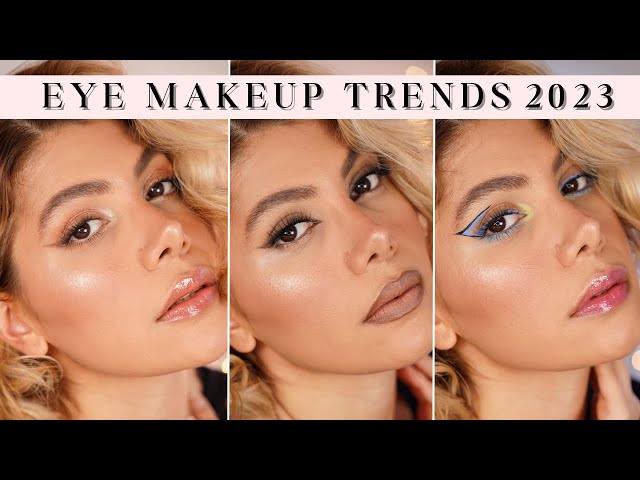The advertisement features three close-up photographs of the same woman showcasing distinct eye makeup trends for 2023. The image is framed with black bars at the top and bottom, creating a letterbox effect. Across the top, a white band with bold, serifed text that reads "Eye Makeup Trends 2023" in black, creating a striking 3D shadow effect, introduces the theme.

In the left photograph, the woman, a white female with dark brown eyes, sports a subtle look with pinkish gloss on her lips and a slight reddish hue on her eyelids. Her dark eyeliner creates a delicate emphasis on her eyes, which gaze directly forward. Her wavy blonde and brown hair frames her face from above, creating a soft, natural effect.

The middle photograph offers a more dramatic, smoky look with a cat-eye effect. Her lips, now a brownish beige nude, draw less attention, allowing the focus to remain on her eyes, which are accentuated with darker, smokier eye shadow. Her gaze remains direct but less upwardly tilted than in the first image.

The right photograph features the boldest look with blue and black eye makeup. There’s a distinctive blue triangle on her right eyelid, with additional blue shading around the eyes and black outlines enhancing the dramatic effect. Her lips are glossy with a reddish tint, complementing the vivid eye makeup. Her hair remains consistently styled across all images, emphasizing continuity despite the varied makeup styles.

Overall, the advertisement effectively highlights the versatility of eye makeup trends using the same model and similar angles to demonstrate the range of looks achievable.